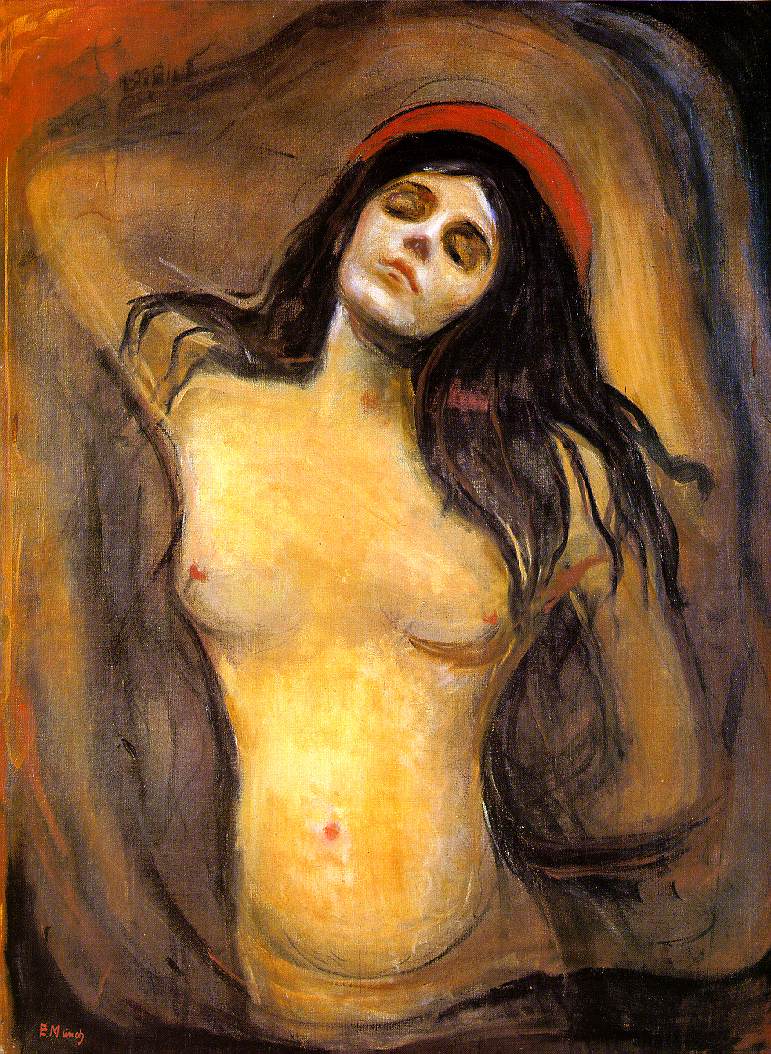This oil painting depicts a young, unclothed woman against a mottled backdrop of brown and black shades. The woman's head is tilted back with her eyes closed, and she exudes an air of calm and repose. Her long, dark shoulder-length hair cascades down, while a vibrant red, halo-like curve or scarf encircles the top of her head. She has a distinctly flesh-colored complexion with hints of orange, and her breasts with red nipples and a swollen belly with a red belly button are exposed, suggesting potential pregnancy. One arm drapes behind her waist, while the other is positioned behind her head. The composition includes bands of brown paint surrounding her, adding to the textured depth of the scene. The painting is marked with a red signature on the bottom left, although it is too small to be legible.